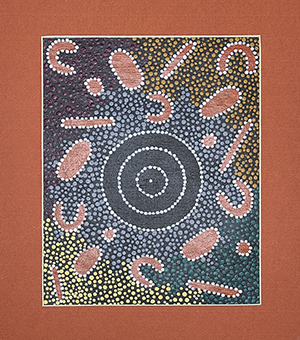The artwork features a rust-colored rectangular background serving as a matte. The primary image is slightly rectangular and predominantly rendered in blue hues. Dominating the center is a meticulously designed circle comprised of concentric rings: three black circles enclosed by white bead-like accents, culminating in a white bead at the very center. Surrounding this central motif are blue dots, which stretch from the center towards the lower right quadrant of the artwork.

In addition to the central design, various shapes resembling microscopic bacterium are scattered throughout. These shapes are brown with white dots and come in different forms, including oval, backwards C-shaped, and rod-shaped figures. The upper right corner of the piece features tan-colored dots, while the lower left corner transitions into yellow-colored dots, adding a gradient-like effect to the detailed composition.